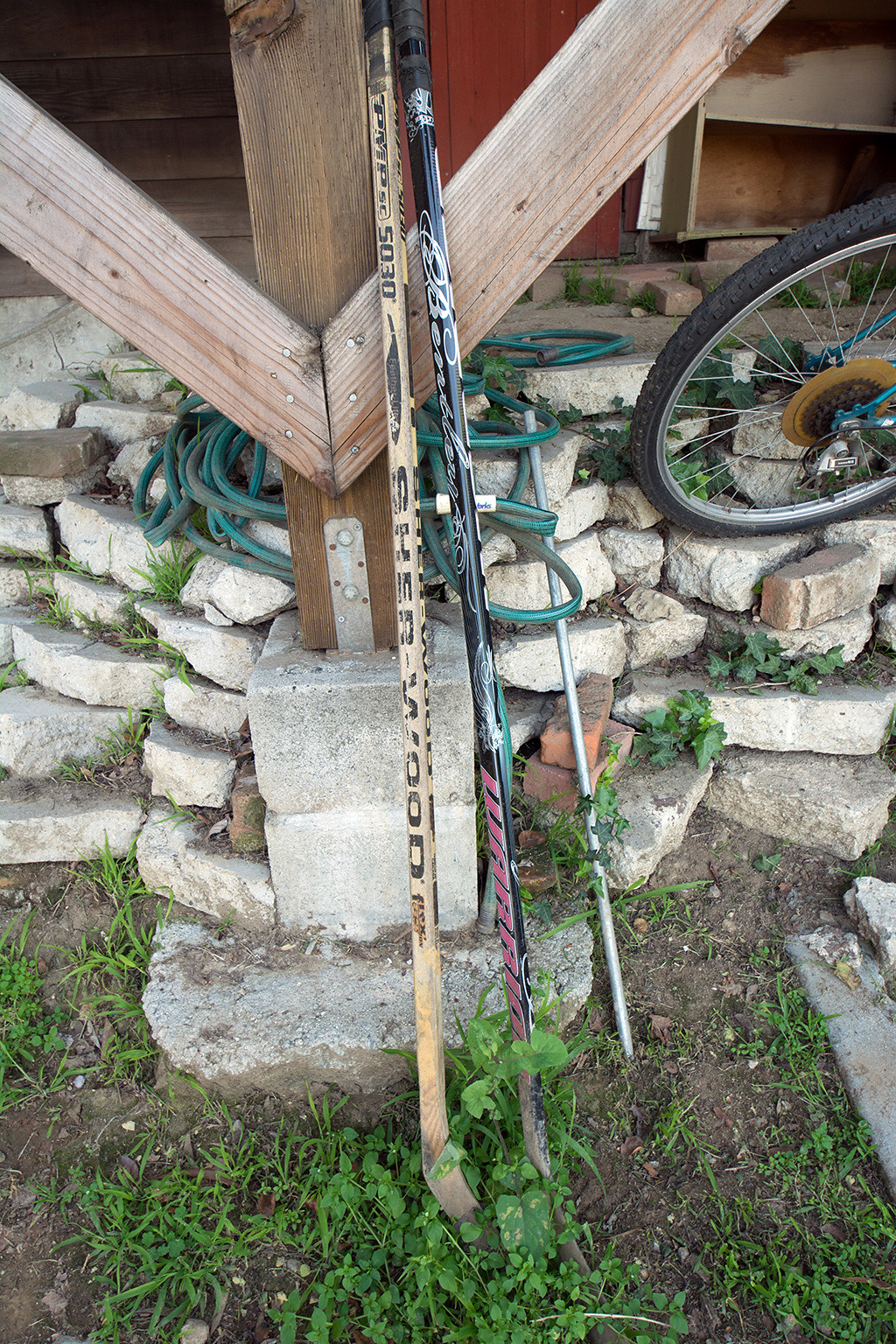The image captures a scene outside a house, likely near a porch or balcony, during the day. Dominating the foreground is a wooden support beam connected to a concrete post, which is part of the structure's foundation. The beam rises from the ground and is reinforced diagonally by two additional wooden beams. Leaning against this beam are three objects: two hockey sticks and what appears to be a metal rod or stick, partially stuck in the ground. The first hockey stick is natural wood, bearing the brand name "Sherwood" and the number "50-30" on its handle, while the second is black with red text at the bottom and white writing at the top.

Grass and dirt cover the ground at the base of the beam, blending into the surrounding area which includes loose rocks and stone pavement. A green garden hose lies coiled behind the post. To the right side of the beam, the back tire of a bicycle, possibly dark turquoise in color, sits atop the rocky ground. In the background, there is a stack of light tan and off-white boulders forming a wall, and beyond this, the outer wall of the house is visible, composed of brown wood with a shelf that appears rickety and warped. The overall ambiance suggests a rustic, possibly cabin-like environment.